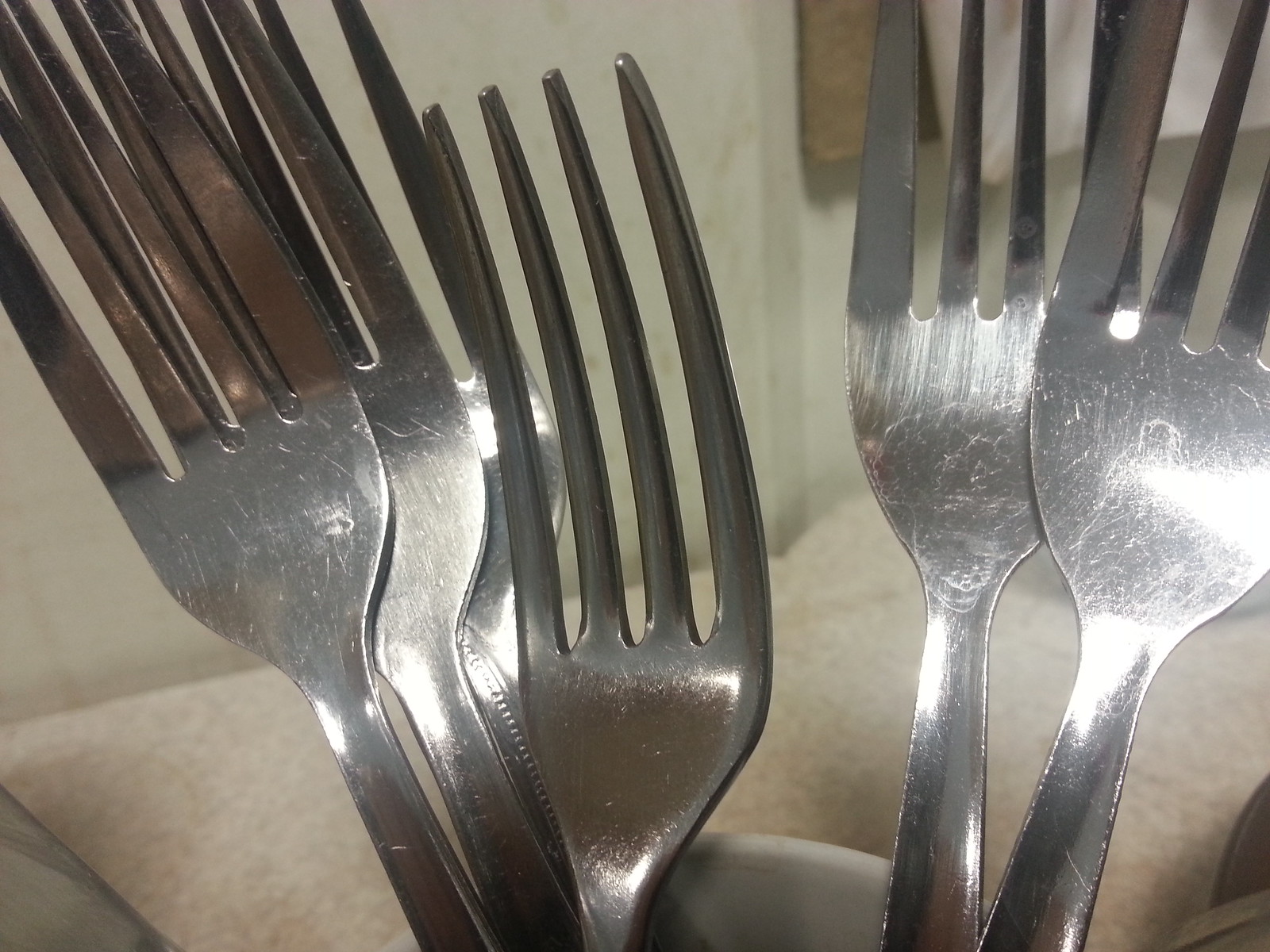In the image, six identical, high-polished stainless steel forks with four prongs each are positioned against a light-colored background. The forks are only visible by their tines, which reflect light, giving them a shiny appearance. They are placed on a white ceramic cup situated on a tan Formica counter speckled with white. Behind the forks, there is a light-colored piece of fabric, possibly a towel, hanging on a painted wall. Subtle hairline scratches and buff marks can be seen on some of the forks due to the close-up nature of the photograph and the gleaming reflection of the light.